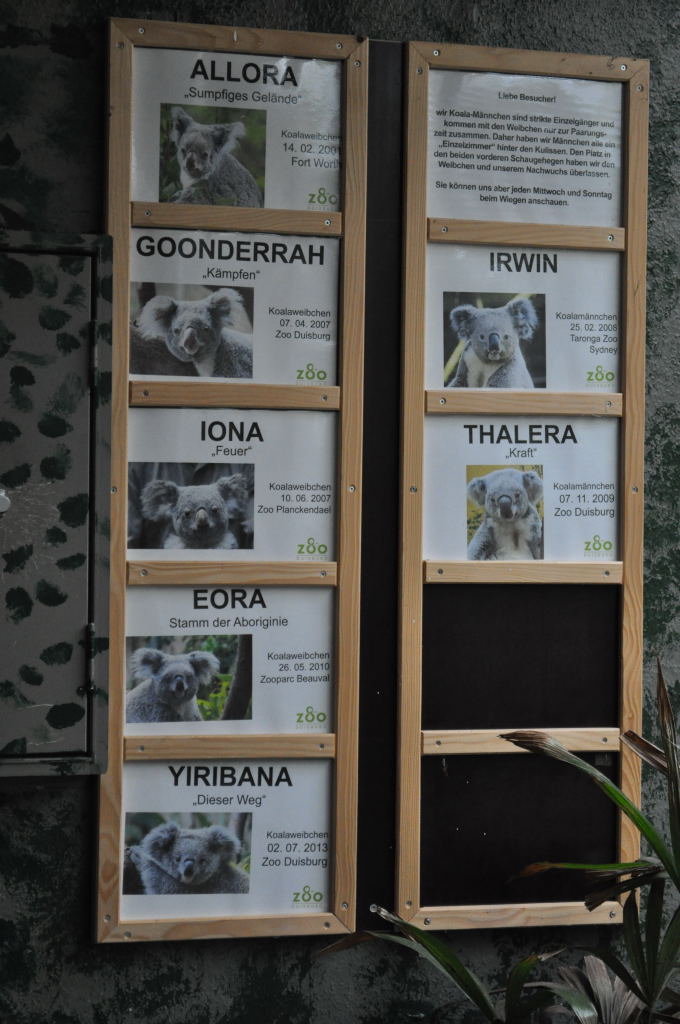This is a color photograph taken outdoors, likely at a zoo or a koala rescue center. The image shows two wooden display frames attached to a wall, each divided into five sections. Each section contains a sheet of paper featuring a black and white mugshot of a koala, accompanied by the animal's name and information. The left frame presents five koalas: Allora at the top, followed by Gundera, Iona, Eora, and Yiribana. Each koala's section includes additional details, possibly including a nickname or location, which may be in German. The right frame has a sign at the top that is not fully legible, and contains photos of two koalas: Erwin and Thalera, with the bottom two sections left blank. Positioned on the ground in front of the right frame is a potted green plant adding to the naturalistic setting. The overall setup suggests it is an informational sign designed to educate visitors about the resident koalas.